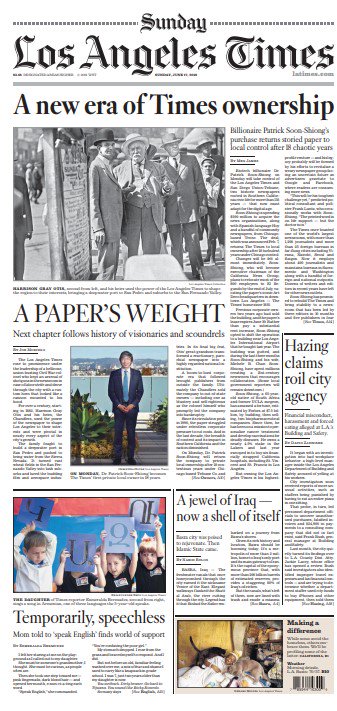In this image, we see the front page of a newspaper laid out against a solid white background. At the very top center is the word "Sunday" printed in black text, flanked by lines of small dots extending to the left and right edges of the page. Below this, the masthead displays "Los Angeles Times" in black and gray text, followed by "latimes.com" in a smaller font. A thin gray horizontal line separates the masthead from the main headline area.

The prominent headline reads, "A new era of Times ownership: billionaire Patrick Soon-Shiong's purchase returns storied paper to local control after 18 chaotic years." Lower down, sub-headlines, though small and slightly blurred, hint at an overarching theme. One such sub-headline reads, "A paper's next chapter follows history of visionaries and scoundrels."

Further down the page, there's an additional article titled, "Temporary Speechless: Mom told to speak English finds world of support," accompanied by an image of a man in a dark suit, white shirt, and blue tie. The text within this image is small, making finer details difficult to discern, but the overall layout effectively captures reader attention through a mix of visual and textual elements.